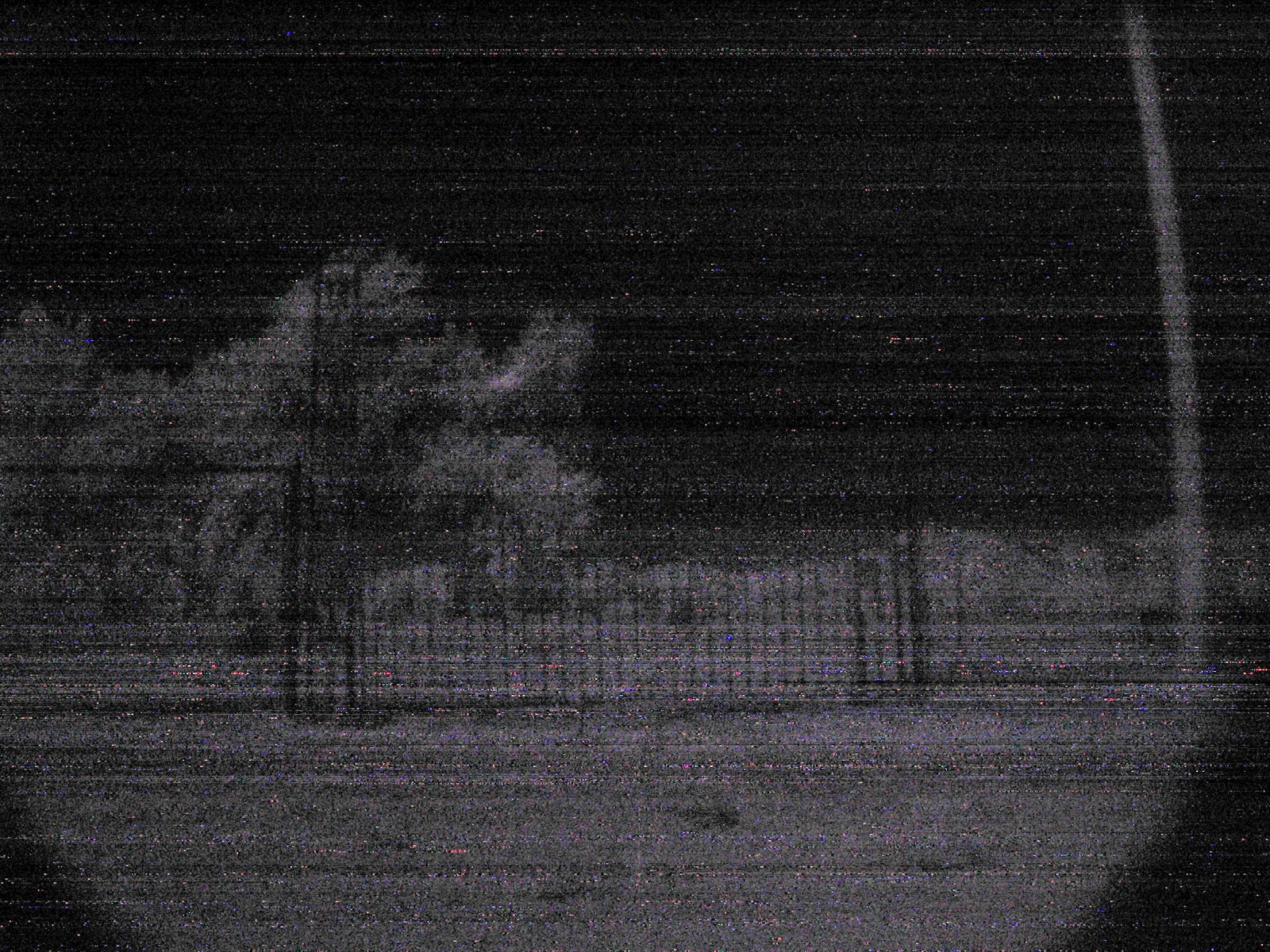This black-and-white image has the appearance of a pixelated view reminiscent of an older digital screen. In the foreground, a white-shaded area dominates, except for the bottom corners, which are black. This creates a triangular, rounded partition at the bottom. A fence stretches horizontally across the image, and to the left, a few trees are distinguishable. On the right stands a light pole extending upwards, from which an electricity wire stretches horizontally across the scene. The sky above is an expanse of black, interspersed with fine, linear shading, hinting at techniques like pointillism or grainy graphics. Upon closer inspection, the image reveals a speckling of tiny pink, yellow, and blue dots, imparting a subtle sense of color that predominantly appears black-and-white from a distance. The overall composition evokes a sense of digital nostalgia and abstract art.